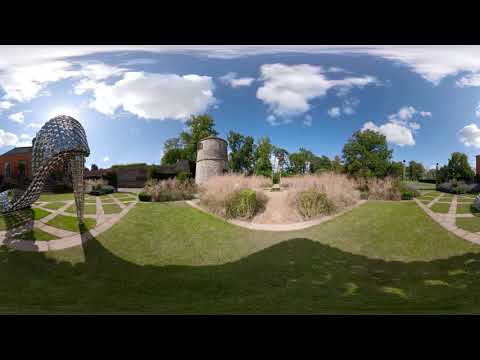The image depicts a well-manicured park or garden, framed in a vertical and rectangular shape. At the very top and bottom, there are black horizontal stripes, enhancing the focus on the central photograph. The landscape features a sprawling green grassy area, meticulously mowed, with various light tan brick or concrete walkways crisscrossing through it. The pathways form intricate patterns, including gray-stone diamonds filled with green grass. In the middle of the scene, there is a circular area where the grass appears taller and brown, possibly indicating out-of-season flowers, and a small black plaque that’s unreadable from this image.

A striking element on the left side is a large, silver metal sculpture in the form of a high-heeled shoe, webbed and towering at least one story high. On the far left, a stone tower, possibly two stories tall, adds to the garden's artistic and structured ambiance. Behind these features, a row of trees stands under a vivid blue sky adorned with white, puffy clouds that seem to stretch and warp towards the edges, lending a surreal touch to the overall image.